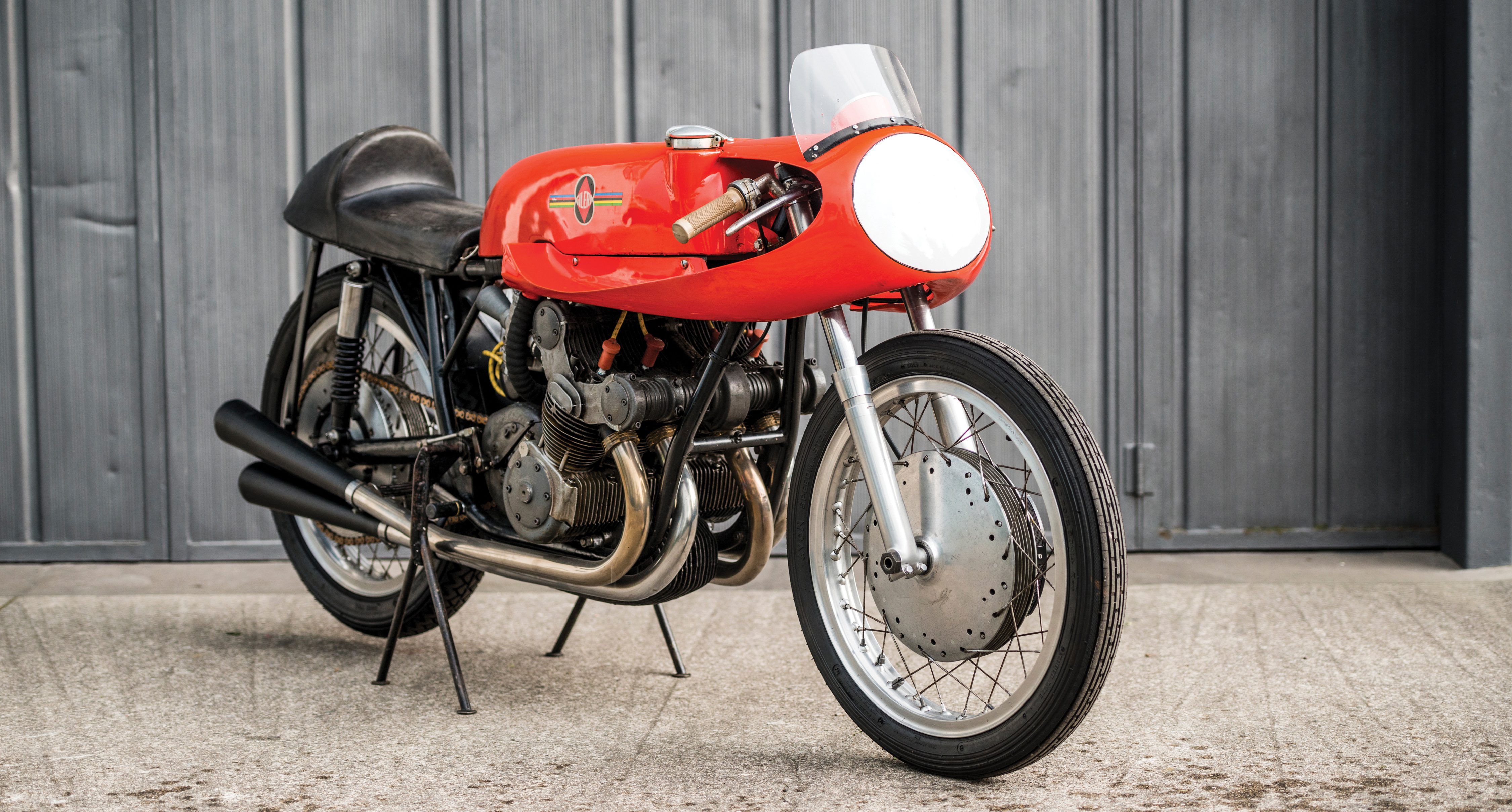This photograph captures an intriguing, vintage-styled motorcycle parked inside a garage. The bike features a compact frame with an old-model design, characterized by a notably small motor housing. The body of the motorcycle is predominantly red on the top with a stark contrast provided by black tires, a black seat, and silver-colored rims. A modest visor or windshield guard is mounted at the front.

The motorcycle is supported by two kickstands, one on each side, ensuring its stability. It also sports dual exhaust pipes on both sides, enhancing its classic appearance. An interesting modification is evident where the handlebars would normally be; instead, a large, red flashlight-like structure is installed, giving it a unique and somewhat quirky look. The handlebars are now positioned unusually low, contributing to the bike’s unconventional aesthetic. Overall, this modified bike stands as a curious blend of retro elements and peculiar alterations, making it a standout piece in the setting of a dimly lit, cluttered garage.